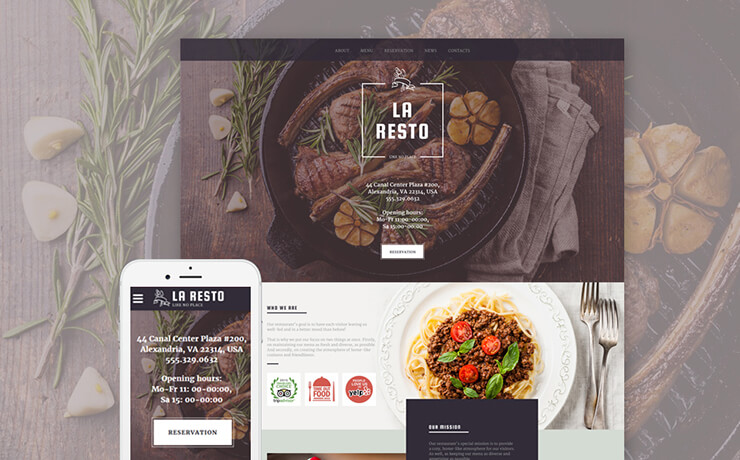This image is an advertisement for a restaurant named LARESTA. At the top of the page, enclosed in a white box, the restaurant's name "LARESTA" is prominently displayed in bold, capital letters. Below the name is the address: "44 Canal Center Plaza, Suite 300, Alexandria, VA," followed by the USA zip code and a phone number. Although the text is somewhat hard to read due to the low resolution and small font size, these details are discernible.

The advertisement lists the restaurant's opening hours, spanning Monday through Friday, along with specific operating times for Sunday, though the exact times are difficult to make out. Beneath the operating hours, a white button labeled "Reservations" suggests an option for making bookings.

Background imagery features a striking photograph of a black pot containing several pieces of steak attached to long bones, accompanied by what appears to be garlic cloves or possibly fruit, garnishes, and other culinary elements. The pot sits atop a brown tabletop, further adorned with assorted garnishes.

In the bottom left corner of the image, there is a phone interface displaying the same details summarized above. Adjacent to the main image, on a white section of the page, there's a picture of a pasta dish accompanied by forks on the right side. The left side features text describing "Who We Are," which offers more insight into the restaurant's identity and ethos. Overall, the detailed depiction aims to entice viewers with both visual and informational appeal.